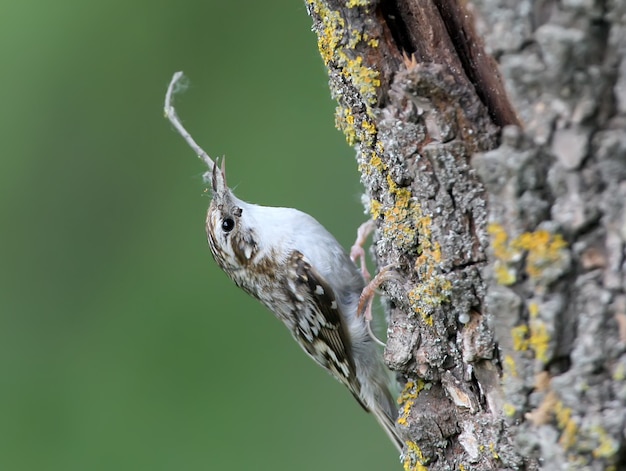The photograph captures a detailed, close-up nature scene of a small bird perched vertically on the trunk of a large tree. The bird, centrally positioned in the frame, displays a white underbelly with brown and dappled gray feathers. Its right eye, black with a white highlight, is wide open as it gazes upward. The bird holds a long, white worm or slender creature in its slightly open beak. It is perched on the grayish bark of the tree, adorned with patches of yellow moss. The background is a hazy, diffused green, setting a natural, tranquil atmosphere. The bird's feet are gripping into the crevices of the tree bark, further emphasizing the intricate details of this vivid wildlife moment.